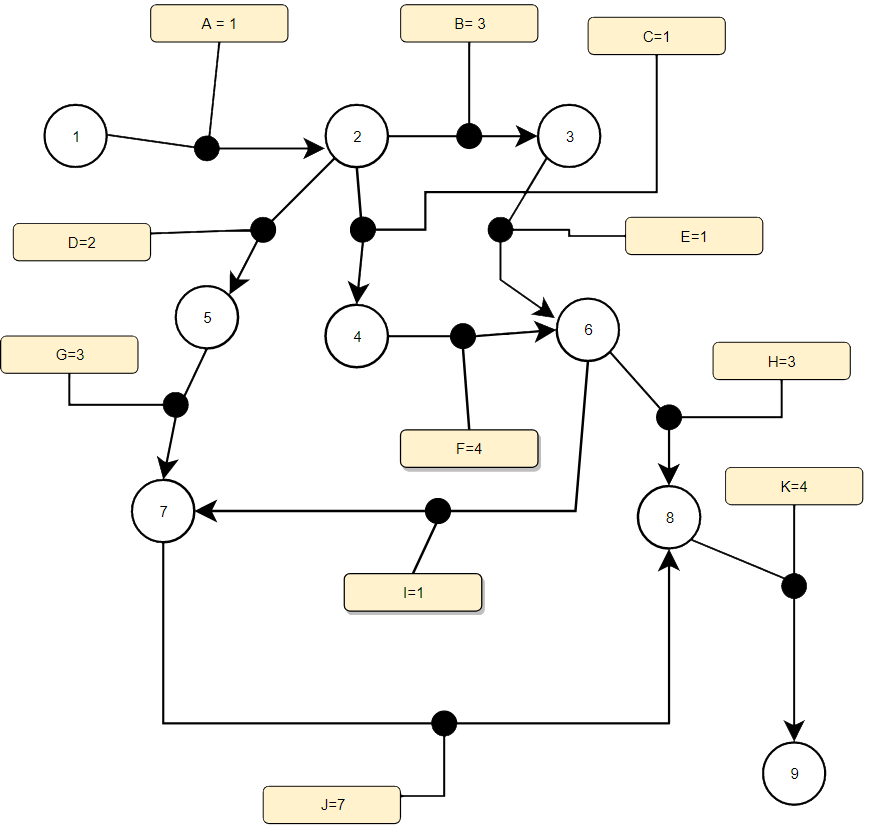This image depicts a detailed black-and-white flowchart schematic, featuring various black dots interconnected by arrows. The diagram is methodically organized, showcasing a sequence of events or processes. Central to the schematic are a series of numbered circles labeled 1 through 9, arranged in order from left to right and top to bottom. 

Adding visual emphasis, several square boxes are shaded in pink and contain specific alphanumeric labels. These pink boxes are systematically positioned throughout the chart. Here's a breakdown of their placements:

- In a left-to-right and top-to-bottom order, the pink-shaded boxes are labeled as follows: 
  - A = 1
  - B = 3
  - C = 1
  - D = 2
  - E = 1
  - G = 3
  - H = 3
  - 4 = 4
  - K = 4
  - 1 = 1
  - J = 7

Each pink square is connected to a solid black dot, indicating a specific step or element within the flowchart. The nature of the diagram suggests it could be representing either a complex mathematical process or an electrical circuit, though the exact purpose remains somewhat ambiguous. The entire schematic is set against a plain, white background, providing clear visibility to its intricate design.